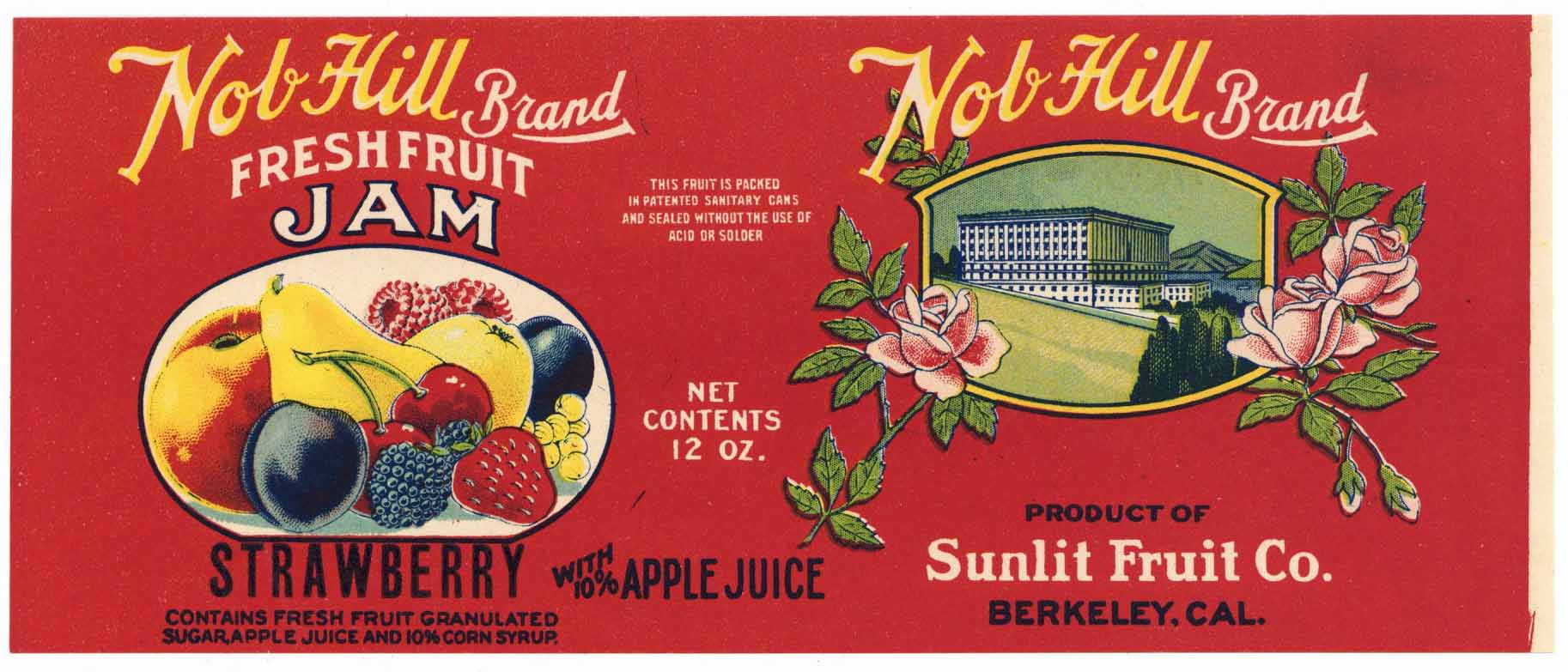This detailed label, originating from a jar of jam, has been removed and laid flat, displaying both its front and back sides. The left side of the label features a vivid red background with the brand name "Knob Hill" prominently written in yellow cursive lettering. Below it, in regular white text, the label reads "Brand Fresh Fruit Jam." Central to the design is a colorful collage of various fruits, including blueberries, strawberries, cherries, peaches, pears, lemons, plums, raspberries, blackberries, and grapes. Beneath this vibrant imagery, the label specifies "Strawberry" in black letters, followed by a list of ingredients: "contains fresh fruit, granulated sugar, apple juice, and 10% corn syrup."

Transitioning to the right side, the label again highlights the "Knob Hill Brand" in yellow cursive and white text. An image of a white building with blue trim, likely their processing center, is set against a scenic green hill with trees. Flanking this image are three pink roses with green stems and leaves—one on the left and two on the right. Below this picturesque scene, the label contains crucial product information in white text: "Product of Sunlit Fruit Company, Berkeley, California," along with details about the jam being packed in patent sanitary cans and sealed without the use of acid or solder, ensuring its 12-ounce contents include 10% apple juice.